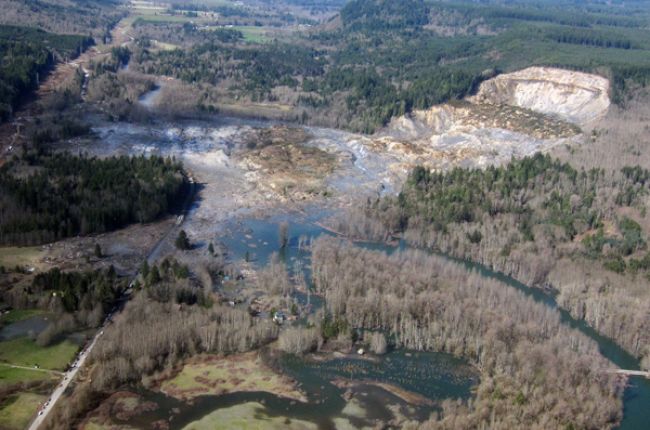An expansive aerial view of a rural wilderness area features diverse landscapes, with green and brown vegetation, water bodies, and distinct natural formations. Central in the frame is a marshland interwoven with multiple waterways, reflecting a blue, partly cloudy sky. Surrounding the marsh are patches of green and brown shrubbery, some live trees, and some dead, grey trees possibly due to flooding. To the left, there's a road running alongside a river with visible cars, indicating a remote, non-urban setting. In the background, lush green trees and grass create a vivid contrast to the barren, deforested or mined area on the right, characterized by white and tan, possibly eroded, earth. At the top right, a possibly man-made, rustic-looking structure resembling a dam oversees water flowing into the lake below, suggesting human interference in the otherwise natural setting.